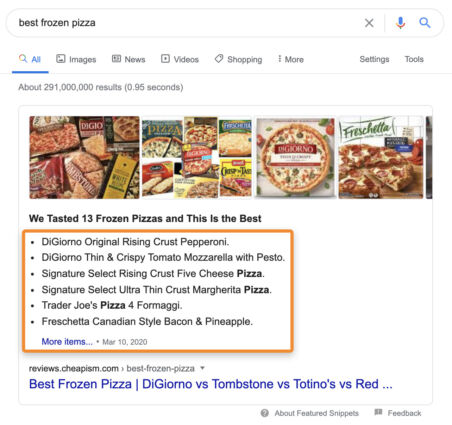In the image, a Google search result page is displayed. At the top of the page, the search query "best frozen pizza" is visible in the search bar. Next to the search bar on the right, there are icons for closing the search (an X), using a voice search (a microphone), and initiating the search (a magnifying glass).

Directly below the search bar are various categories like "All," "Images," "News," "Videos," "Shopping," and "More," towards the left, and "Settings" and "Tools" towards the right. Under these categories, it indicates there are approximately 291 million search results found in 0.95 seconds.

The first part of the search results includes images of different frozen pizza brands and styles. Following these images, in black text, it reads, "We tasted 13 frozen pizzas, and this is the best." Featured prominently in an orange rectangle are:
- DiGiorno Original Rising Crust Pepperoni
- DiGiorno Thin and Crispy Tomato Mozzarella with Pesto
- Signature Select Rising Crust Five Cheeses Pizza
- Signature Select Ultra-Thin Crust Margherita Pizza
- Trader Joe's Pizza 4 Formaggi
- Freschetta Canadian Style Bacon and Pineapple

Below this orange rectangle, in blue text, it says "More items." The date "March 10th, 2020," is written in gray just below.

The first search result is a link to "reviews.cheapism.com," indicated in blue, with the title partially visible as "Best frozen pizza: DiGiorno vs. Tombstone vs. Totino's vs. Red..." All elements of the search result page are set against a clean, white background.